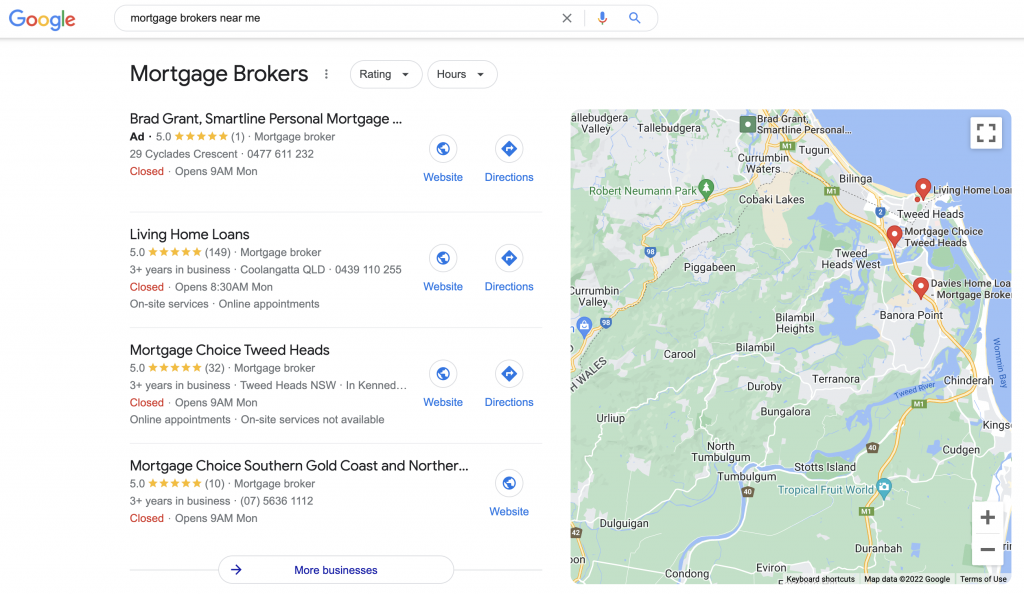This image is a detailed screenshot of a Google search page focused on finding mortgage brokers nearby. In the top left corner, the iconic Google logo is prominently displayed. Adjacent to the logo is the search bar containing the query "Mortgage Brokers Near Me." Within the search bar, there are options to clear the search with an 'X', initiate a voice search with a microphone icon, or start a new search with a magnifying glass icon.

Directly below the search bar, the screen is divided into two sections. On the left side, the heading "Mortgage Brokers" is visible, accompanied by two filter options: "Ratings" and "Hours." Below these filters, a list of mortgage brokers is presented. The first listing is a paid advertisement for "Brad Grant Smart Line Personal Mortgage." Following that, the first non-ad business is "Living Home Loans," then "Mortgage Choice Tweed Heads," and lastly "Mortgage Choice Southern Gold Coast and Northern..." with the rest of the name truncated. Each listing includes hours of operation, and there's a "More businesses" button at the bottom for additional results.

On the right side of the screen, there is a map illustrating the search area. It features red location pins marking the spots where the mortgage brokers are situated. However, only three pins are visible, possibly due to the ad not being location-specific or the map's zoom level obscuring additional pins. The map lacks enough context to identify the exact area being displayed.